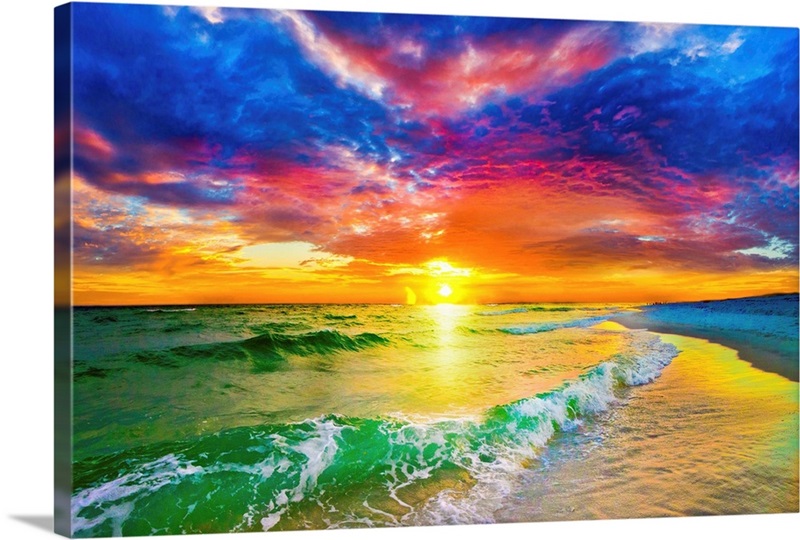This vividly multicolored canvas artwork captures the dynamic beauty of a seaside scene. The focal point is a radiant, bright yellow sun positioned centrally in the sky, which is an extravagant blend of blue, purple, orange, and yellow hues. The sky is dotted with thick, dramatic clouds that add depth and texture to the atmosphere. Below, the ocean is a mesmerizing mix of blue and green, its waves energetically crashing against a golden yellow shoreline. To the right of the canvas, there is an intriguing patch of blue-tinted land, resembling a field of green grass with an unusual blue coloring along its base. This striking representation of nature's elements—sun, sky, sea, and shore—is both captivating and serene.